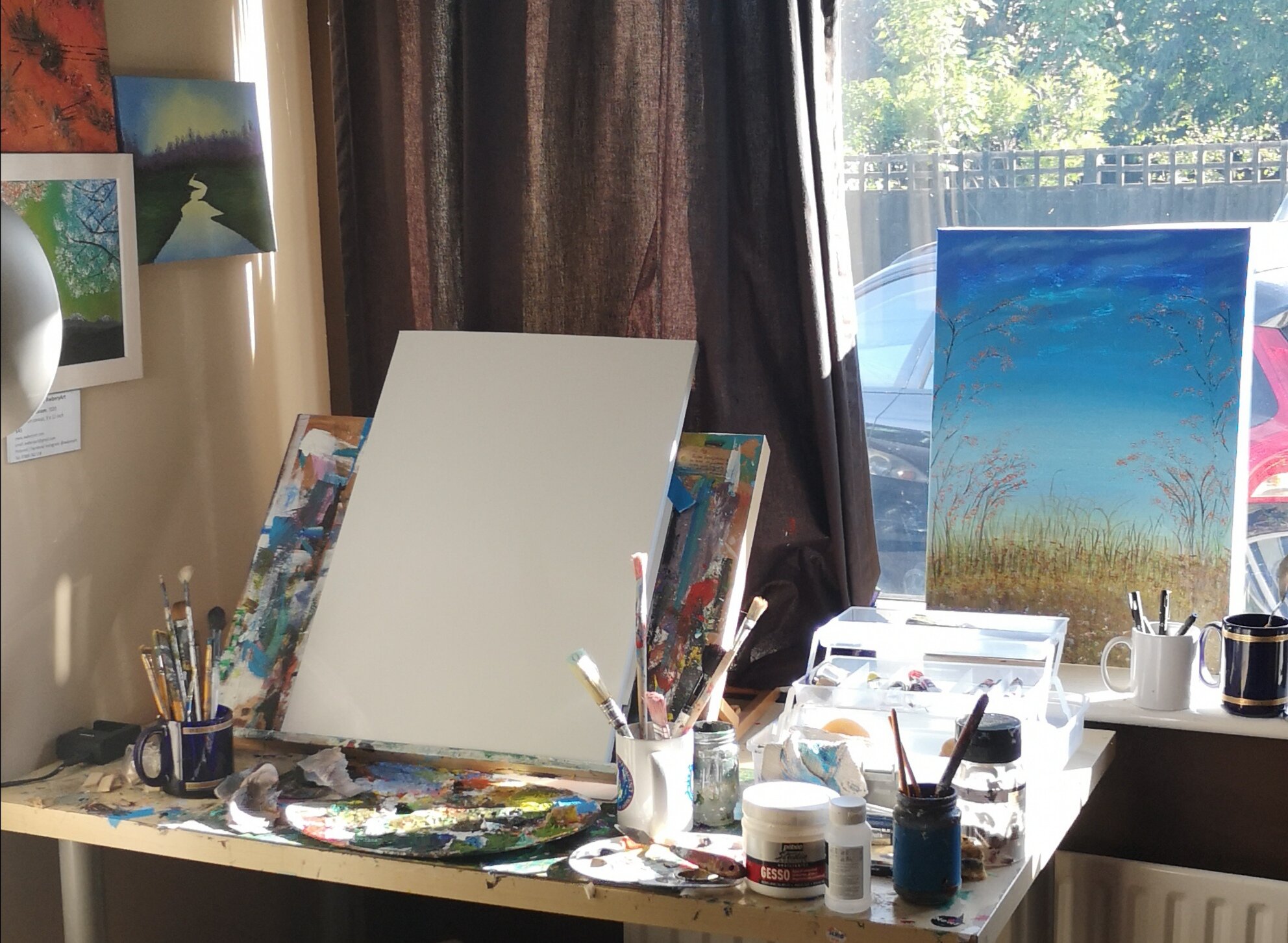This photo captures an artist's room bathed in morning sunlight streaming through a window on the top right. The window offers a view of a backyard with a wooden fence, green foliage, and a couple of vehicles, one black and one red. Dominating the right side of the image is a finished painting depicting a blue sky over a deserted grassy field. In front of this painting, a wooden easel holds a blank canvas, ready for the artist's next project, though no paint is set up on the easel yet. The desk in the foreground is cluttered with paint supplies—including a variety of brushes in two mugs, jars, and smattered paint—highlighting the creative chaos. To the left of the desk, hanging against brown curtains, are additional completed artworks, likely nature-themed, contributing to the room's artistic ambiance.